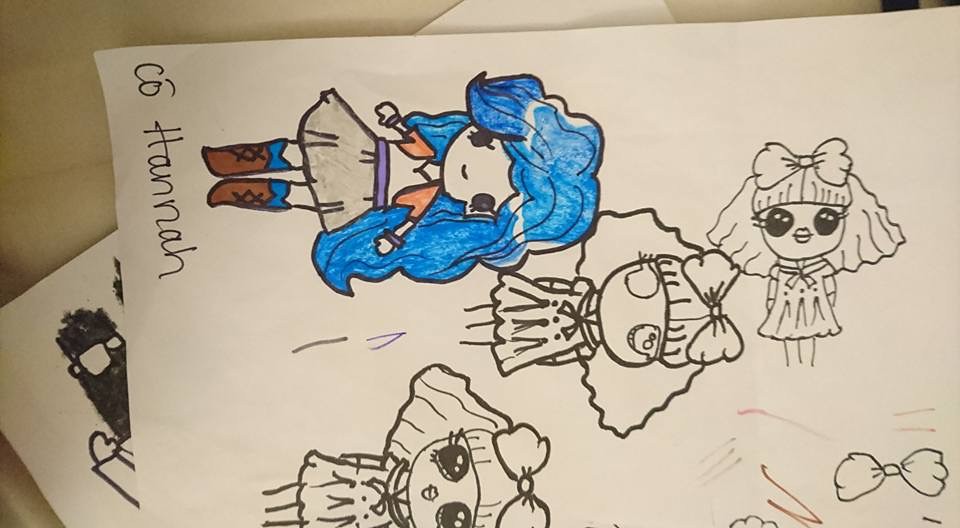This photograph captures two sheets of paper featuring several drawings, partially cropped to show only a part of one sheet. The primary focus is on hand-drawn cartoon characters, distinctly styled as girls. 

One prominent character is a girl with large, expressive eyes and flowy hair that frames her face, extending out to the sides. She is depicted wearing a dress, with her legs visible but her feet cropped out of the frame. This character is consistent across several sketches, and in some, she is adorned with a bow in her hair. These sketches are primarily composed of simple, uncolored outlines.

Another notable character on the second sheet is a similar girl but without a bow in her hair. Unlike the uncolored sketches, this character is fully colored, featuring blue hair, an orange vest, a purple belt, and a gray skirt. Her footwear resembles brown cowboy boots, adding a touch of detail to her attire. Below this colored drawing, there is text that appears to be two words. The first word reads "C-O," possibly with a dash over the 'O,' followed by the name "Hannah." This might suggest the character's name or some contextual detail about her.

Overall, the image showcases a creative display of cartoon characters in varied styles and detail, offering a glimpse into the artist's imaginative process.